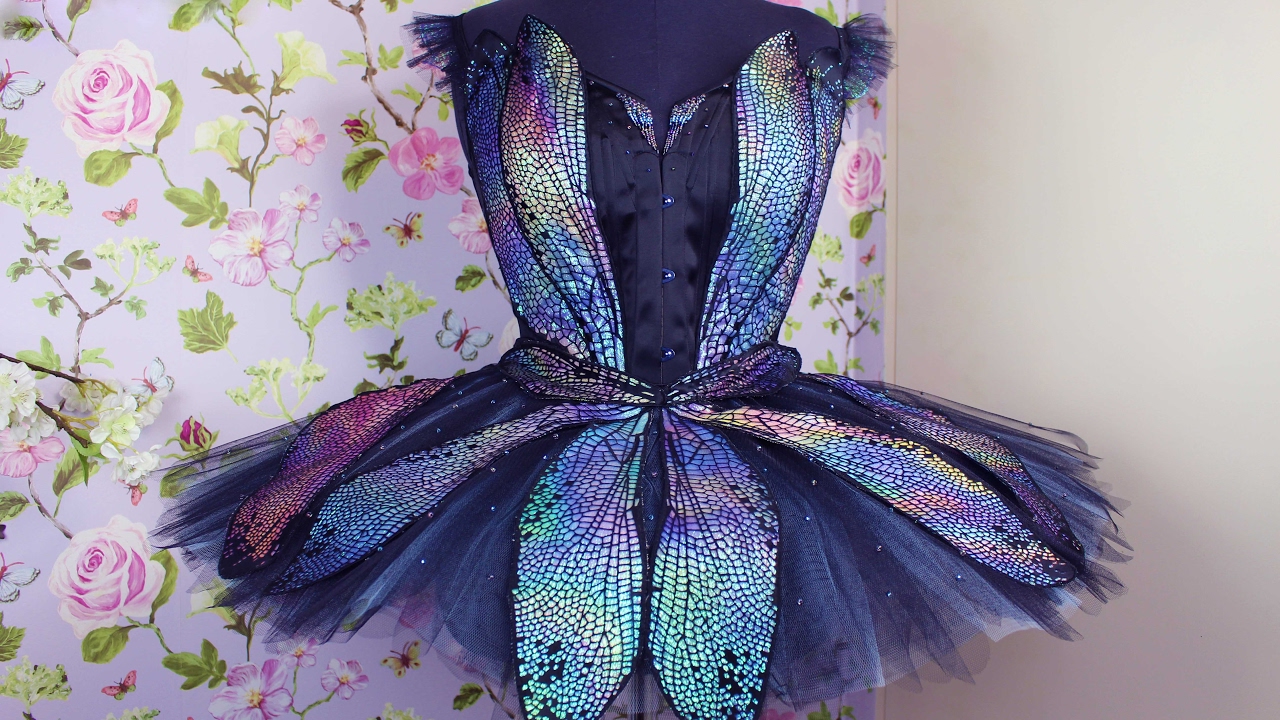This image showcases a striking and vibrant ballerina-inspired dress set against a two-toned backdrop. The left side of the background features a floral pattern with pink roses, green stems, and leafy plants on a purple surface, while the right side contrasts with a plain white wall. The dress, mounted on a dress frame, is an exquisite blend of materials and colors. The bodice, shaped like a vest, is dark blue and features a buttoned element, emphasizing a delicate frill along the shoulders and an open neckline. The skirt mimics the structure of a tutu, composed of multiple layers. The inner layer is a silky black fabric that snaps into place, while the topmost layer resembles translucent, iridescent wings, made of numerous tiny multicolored tiles in shades of purple, light blue, reddish-pink, dark purple, and black. This shimmering, wing-like overlay extends around the tutu, creating an eye-catching, almost ethereal effect, making the dress ideal for a dance routine or costume.